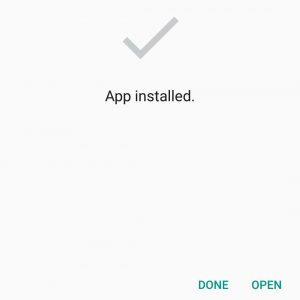The image depicts an installation completion screen, characterized by its simplicity and clean design. Dominating the background is a near-white solid color, subtly differentiated by a very light gray square, adding minimal contrast. Centered at the top of this light gray square is a gray check mark, signifying a successful installation.

Below the check mark, black text reads, "Installation Complete," clearly indicating the status of the process. The simplicity extends to the footer of the screen, where two blue, all-caps hyperlinks are positioned at the bottom right: "DONE" to the left and "OPEN" to the right. These links are presented in a standard hyperlink blue, signifying their interactive nature.

Overall, the screen's design is minimalistic, using just a few colors and elements to communicate the completion of an application installation effectively.